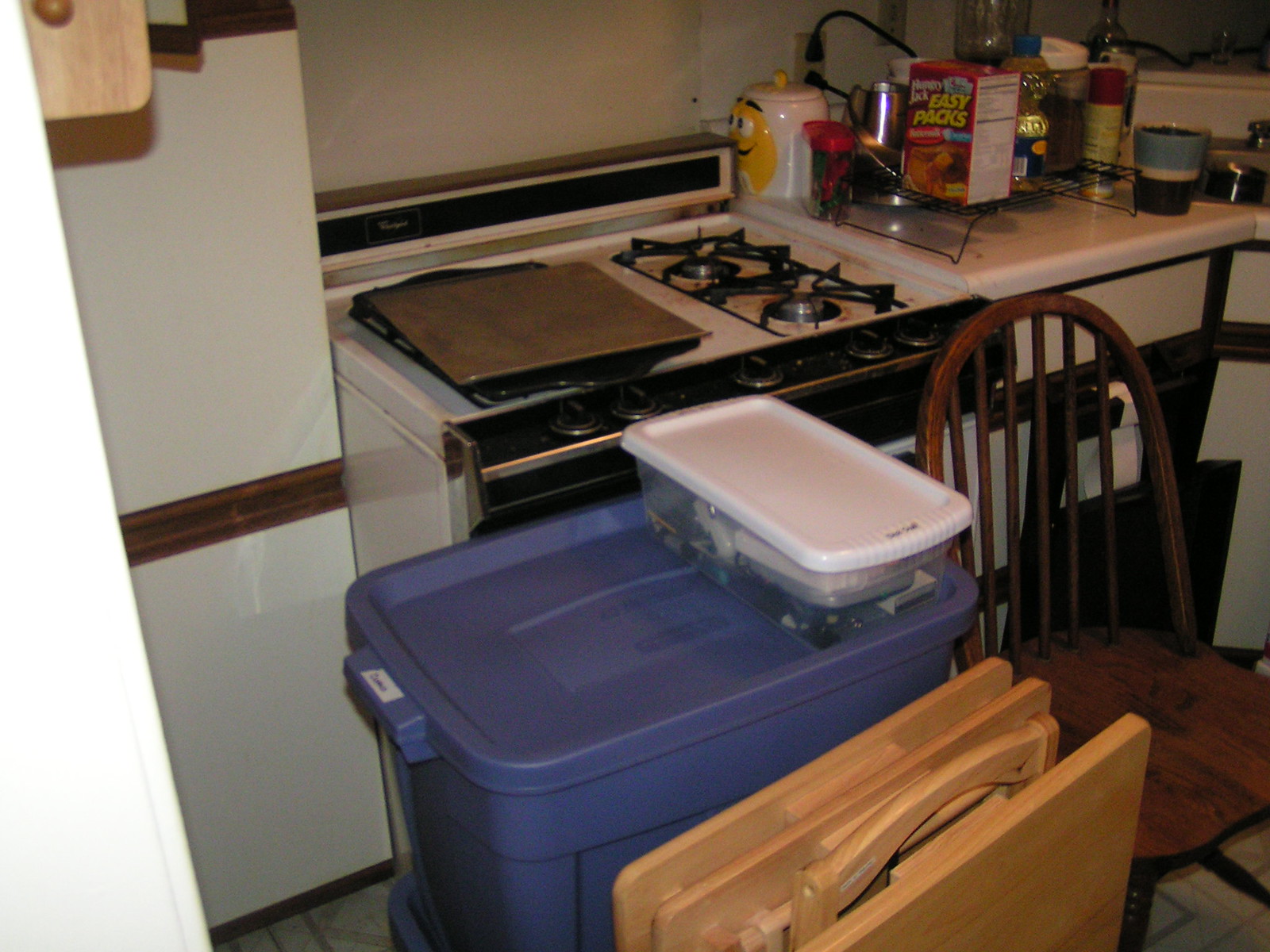The photograph captures a detailed view of a bustling kitchen. On the far left stands a refrigerator, adjacent to which is a free-standing stove with four burners, two of which are obscured by baking trays. Moving right, there's a whimsical M&M cookie jar, a nearby electrical outlet with two plugs connected, and a cookie cooling rack laden with packets and jars of food. The kitchen sink is tucked away in the top right corner, while an array of cupboards line the upper portion of the image.

In the forefront, a brown wooden kitchen chair is prominently positioned. Next to it are two closed blue storage tubs, one bearing a label on its lid. Above these, a clear plastic container with a white lid, also labeled, rests for easy access. In front of these storage containers, there's a brown folding item, which appears to be either a wooden table or possibly foldable chairs. The scene paints a busy, well-used kitchen full of everyday items and storage solutions.